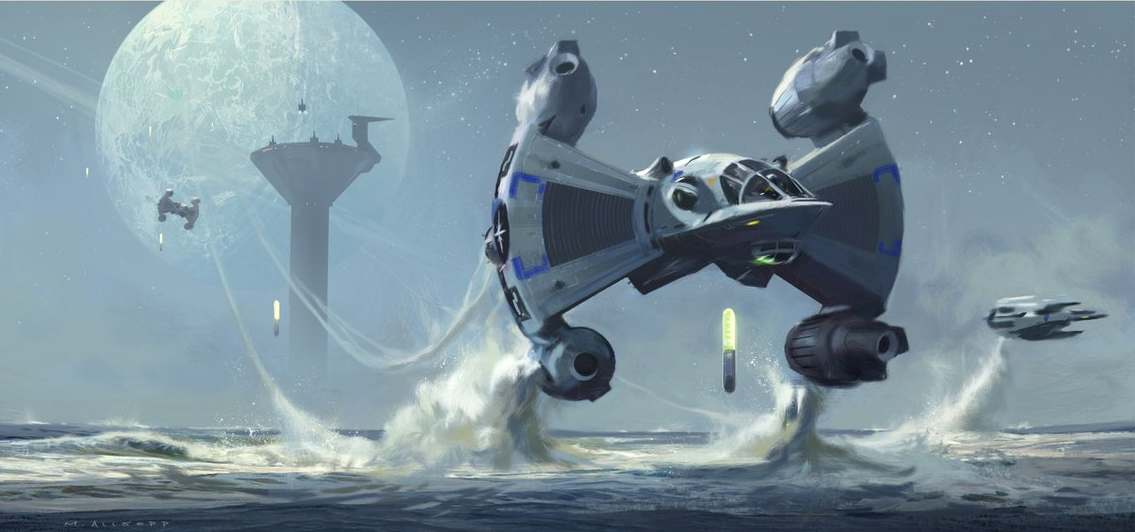This image is a highly detailed digital rendering, resembling a screenshot from a science fiction video game, likely set in the Star Wars universe. The focal point is a dark side TIE fighter, characterized by its distinctive twin triangular wings connected to a central cockpit, which appears silver and black with blue accents. This starfighter skims over a vast ocean, causing dramatic waves and mist from the jet blasts. In the background, a second similar TIE fighter can be seen, suggesting a chase or battle scene. Looming over the scene is a tall white tower which could either be situated on a small landmass or protruding from the water, potentially serving as a launch or docking station for these ships. The sky overhead is a blend of blue and gray hues, featuring a large, luminous moon or planet, adding to the otherworldly atmosphere. The backdrop also includes scattered clouds and distant stars, completing the cinematic and immersive sci-fi aesthetic.